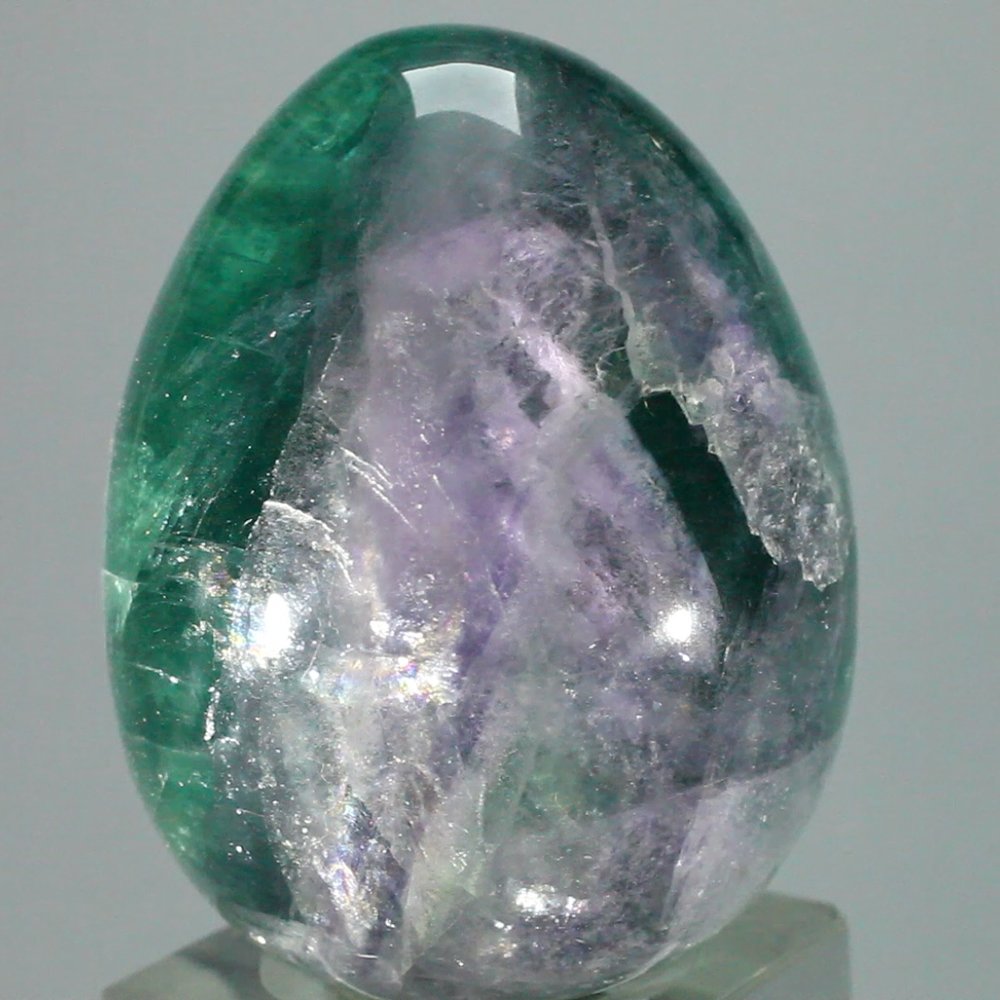The photograph captures a close-up view of a large, polished crystal egg with a sleek, gleaming surface. The backdrop is a subtle grey with a slight greenish hue, enhancing the visual appeal of the egg. The crystal egg is propped on a cube-like base that appears to be made of a clear mineral or plastic. The egg exhibits a gradient of green tints along its left edge, extending over the top and around the right side, which frames a central, whiter area with a cloudy appearance and hints of light purple. Various internal fractures and jagged pieces are visible, radiating from the center in different directions. The egg is highly polished, evidenced by distinct reflections and a shiny glimmer, particularly noticeable at the top and left corners. The intricate mix of multiple green shades, from dark to light, gives the egg a sophisticated and potentially valuable look, similar to an exhibit piece one might find in a museum.